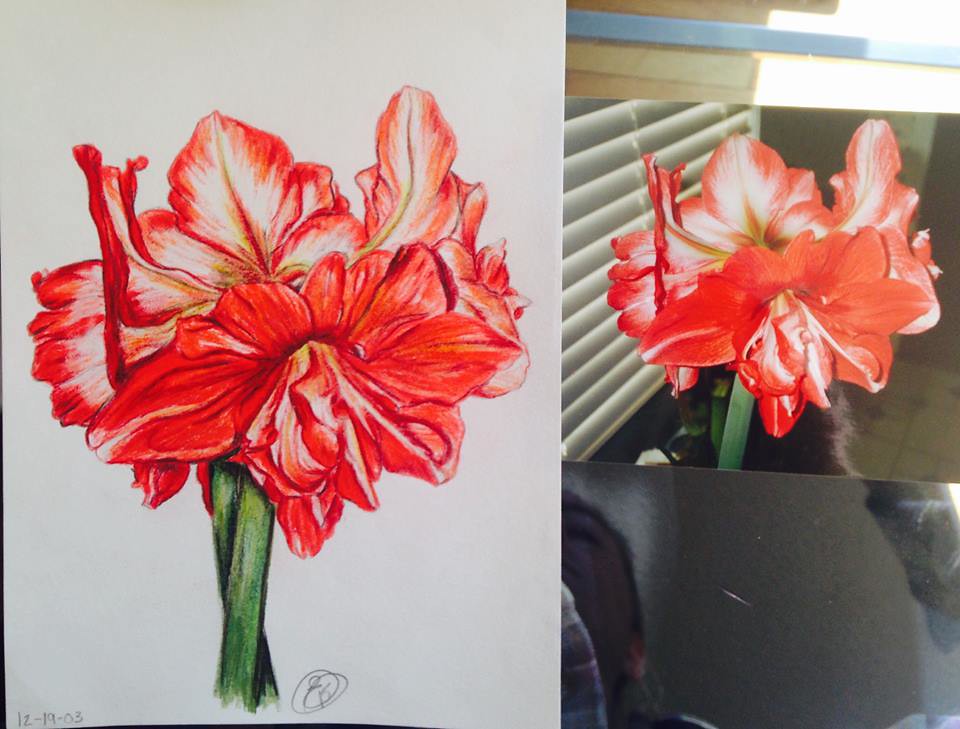This image features two side-by-side pictures: on the left, a detailed drawing or painting of an orange-pinkish flower with intricately designed petals and a green stem, and on the right, a photograph of the same flower taken in real life. The flower in both images has a striking appearance with a large vein that runs down the middle of each petal and white accents radiating from the center. The left-hand artwork appears to be drawn on paper using colored pencils or pastels and is signed with initials and dated "12-19-03" in the bottom left corner. The striking resemblance of colors and details suggest that the real flower, photographed against a backdrop of white blinds and a black rectangular object, served as the model for the high-quality drawing.